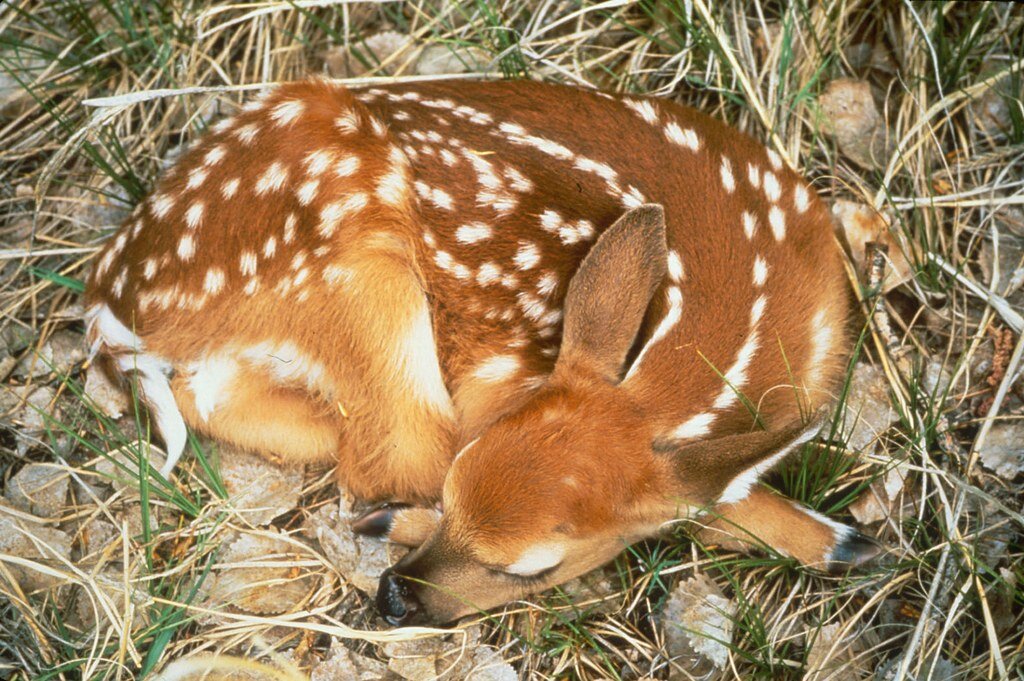This is a stunning, professionally captured close-up photograph of a baby deer, known as a fawn, nestled in a bed of lush green grass intermixed with light brown twigs and small gray rocks. Dominating the center of the image, the fawn is curled up, resting its head on its feet and sound asleep. Its light brown coat features delicate white spots that form two lines, resembling tram tracks, running from its neck to its rear. The fawn’s large, pointy ears, cute black nose, and closed eyes give it an endearing, peaceful appearance. The photograph highlights various shades of brown on the fawn, with darker hues on its back and lighter tones around its legs, as well as a short tail that is mainly white with a hint of brown. The clarity and sharpness of this image suggest a professional touch, capturing the intricate details and serene beauty of the scene.